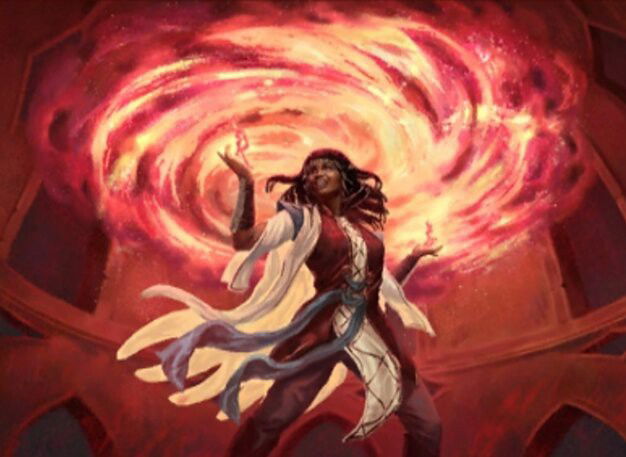The image features a powerful and dark-skinned woman standing confidently in the center of a grand, chamber-like setting, reminiscent of a scene from an animated TV series or a beautifully detailed piece of digital or watercolor art. She has an imposing stance with her legs wide apart and her arms even wider, her hands pointing upwards as if casting a spell. She is adorned in a striking ensemble: a red top with a flowing white centerpiece trimmed in gold, matching purplish pants, and a long, flowing blue cloth attached to her attire, along with flowing white cloth around her arms and gauntlets. Her long, black hair flows around her as she smiles confidently. Above her, there swirls a large fiery twist of bright red, yellow, and orange light, symbolizing energy and magical power, with a large artistic letter "R" hovering just above her right hand. The room behind her, possibly part of a medieval or Renaissance-like building, features peaked door openings and seems bathed in a red hue that complements the fiery glow of her spell.